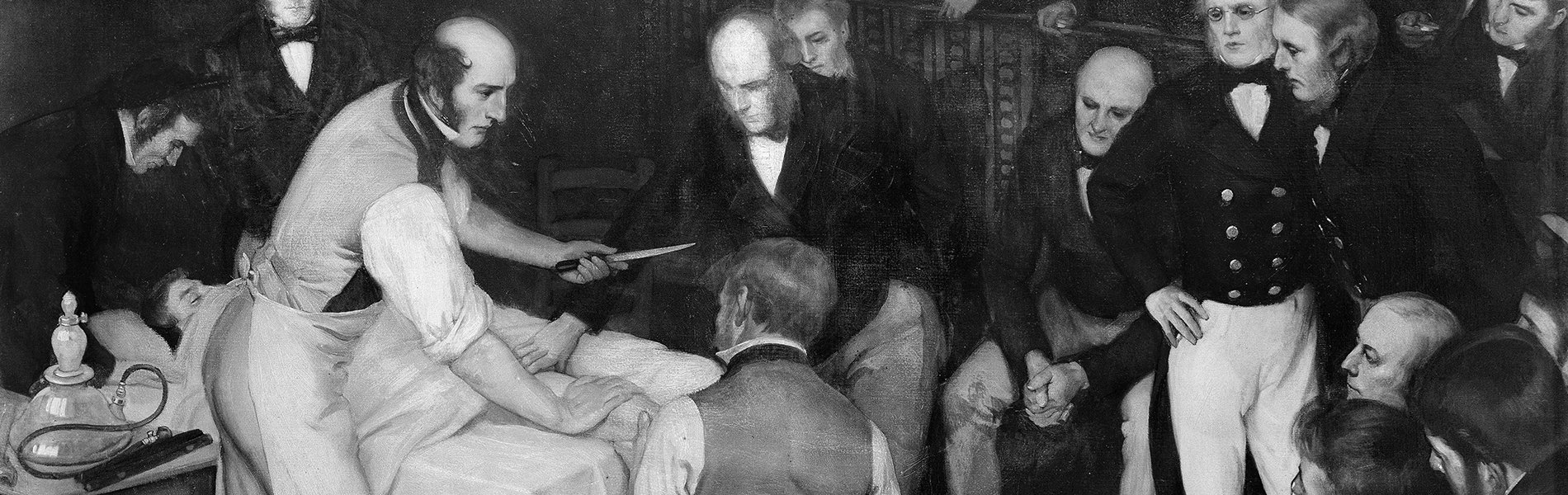In this detailed black and white image, reminiscent of a scene from a couple of hundred years ago, a room full of men dressed in old-fashioned suits and varying facial hair styles centers around a dramatic medical procedure. The focal point is a man lying unconscious on a table, covered by a white sheet, positioned with his head to the left and knees to the right. On the left side of the room, a balding doctor clad in a white shirt and apron stands over the man, holding a knife in his right hand and appearing to prepare for a surgical or autopsy procedure. The doctor is watched closely by another man with his back turned to the camera, who wears a vest and white shirt, and has blonde hair. At the head of the table, two men in black suits hold the unconscious man down, ensuring he remains still. To the doctor's immediate right stands a balding man in a black suit, holding his hands together between his legs, observing intently. Seated to his right, another balding man in a suit watches the scene unfold. Additionally, two men are seen standing close together, leaning in and observing the procedure while dressed in a combination of black jackets and white pants. In the bottom right corner, the heads of three more onlookers are visible, indicating their keen interest in the ongoing situation. The overall atmosphere suggests a medical or autopsy procedure conducted without modern gloves, highlighting the historical setting and the intense focus of the spectators on this dramatic moment.